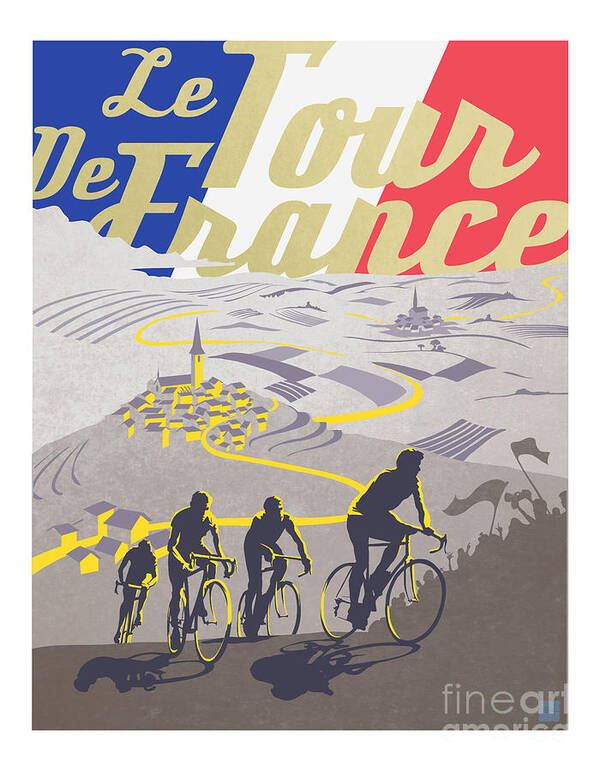This poster, related to the cycling event "Le Tour de France," features a detailed and abstract illustration rich in color and symbolic imagery. The top of the vertical, rectangular poster displays the French flag, with blue on the left, white in the middle, and red on the right. Overlaid on the flag are the words "Le Tour de France" written in gold letters, each word capitalized.

Below the text and flag, the main illustration depicts an evocative scene rendered in grays, blacks, yellows, and hints of blue. The center features a brown path with a subtle yellow road that serpentines through the scene, suggesting hilly terrain and farming fields, ultimately leading towards distant villages. There are two clusters of buildings, one to the right and another upwards along the road, each containing multiple structures with dark roofs and prominent churches.

Four cyclists are prominently featured on the brown path, their silhouettes highlighted in black and yellow to give a sense of movement and light reflection. The cyclists, on road bikes, appear to be racing towards the viewer, with shadows cast and yellowish highlights on their shoulders and one tire. 

Behind the cyclists, a grayish background outlines a townscape with detailed contours of land and buildings. This background seamlessly transitions into a crowd of people, drawn in dark silhouettes, some waving flags, enhancing the event's dynamic and festive atmosphere. This artwork merges fine art with a sports theme, making it a striking and evocative representation of the "Le Tour de France."